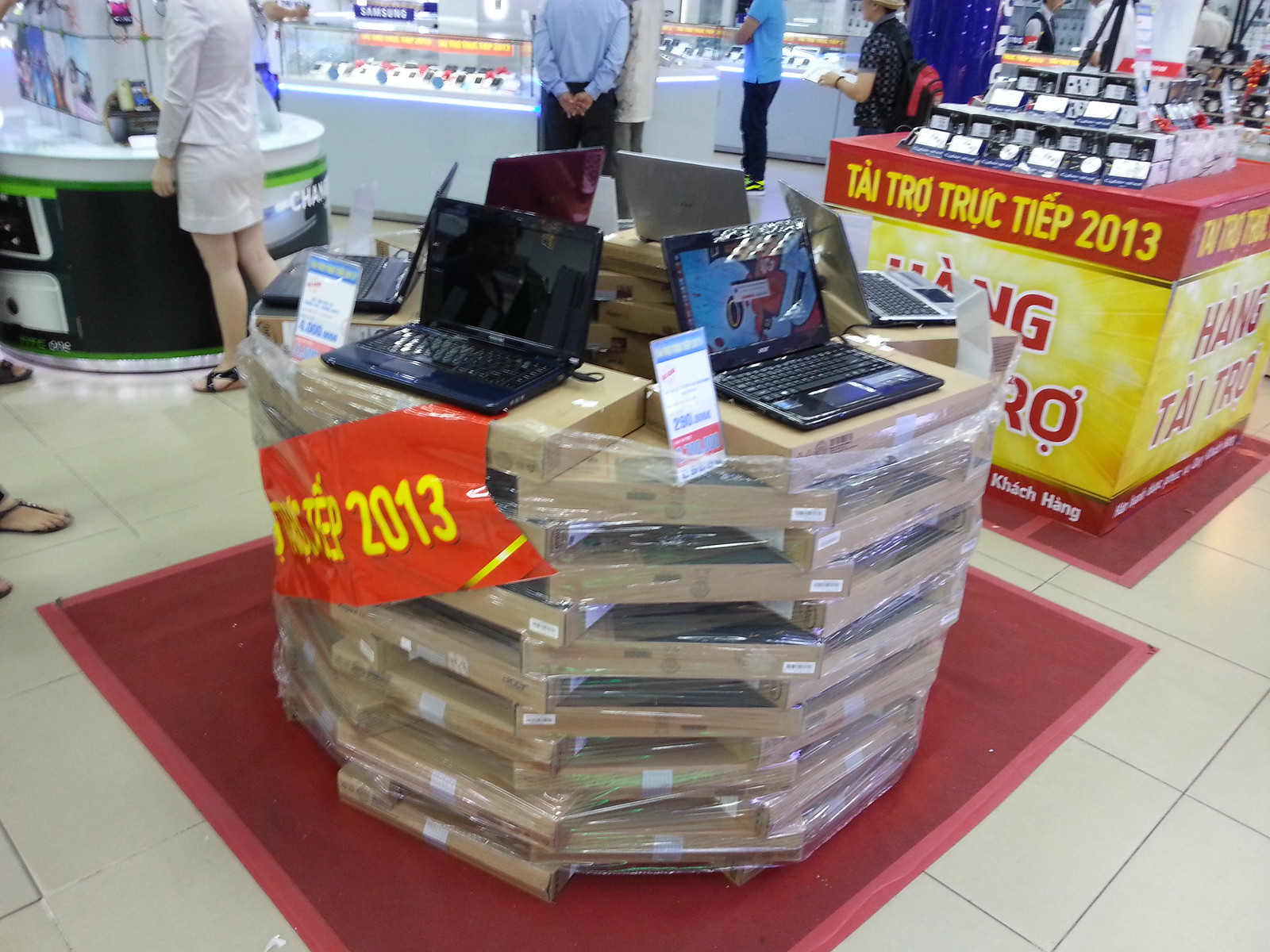This photograph depicts the inside of an electronics store, likely taken in 2013, as indicated by signage. The store appears to be in a foreign country, with some text suggesting it might be Vietnam or Hong Kong. In the background, several display areas are visible, featuring glass-topped counters likely showcasing smartphones or GPS devices. In the foreground to the middle left, a large red square carpet rests atop a brown-tiled floor. On this carpet sits a makeshift table constructed from layered and plastic-wrapped cardboard boxes, about three feet high. Arranged in a circular fashion atop these boxes are six laptops, each black and silver, with accompanying signs displaying product information and prices. The scene includes a mix of employees and customers, with around six or seven people milling about the store.